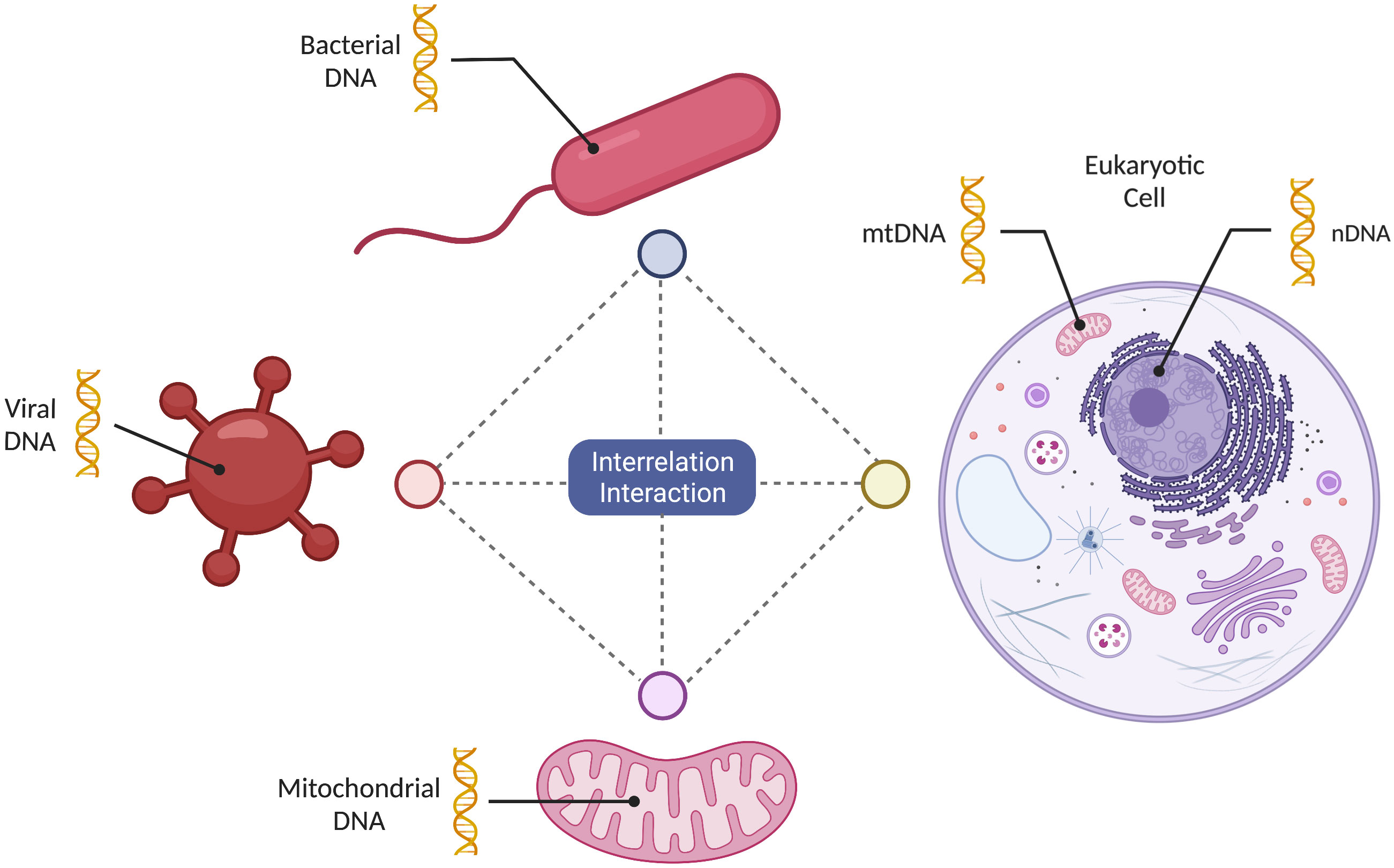The image features a detailed diagram against a plain white background, approximately four inches high by six inches wide, illustrating various aspects of DNA and cellular structures. In the upper left, a yellow strand is labeled as "Bacterial DNA," connected via a black line to a red, rounded rectangle with a red tail. In the left center, a label for "Viral DNA" points to a red circle with smaller red circles surrounding it. At the bottom left, "Mitochondrial DNA" is indicated next to an enlarged pink bean-shaped structure.

Dominating the right side of the image, a light bluish-purple circle with a dark purple outline represents a cell, with "Eukaryotic Cell" printed above in black. Inside this circle, a dark purple nucleus is depicted, along with a pink bean shape connected to a yellow spiral labeled "MT-DNA." Another label inside the circle points to a yellow strand tagged "N-DNA."

Central to the diagram is a diamond-shaped region marked "Interrelation Interaction," with colored circles at its four corners: blue at the top, yellow on the right, purple at the bottom, and pink on the left. The diagram clearly delineates the different types of DNA and their interactions within the cellular context, presented in a well-lit and highly legible manner.